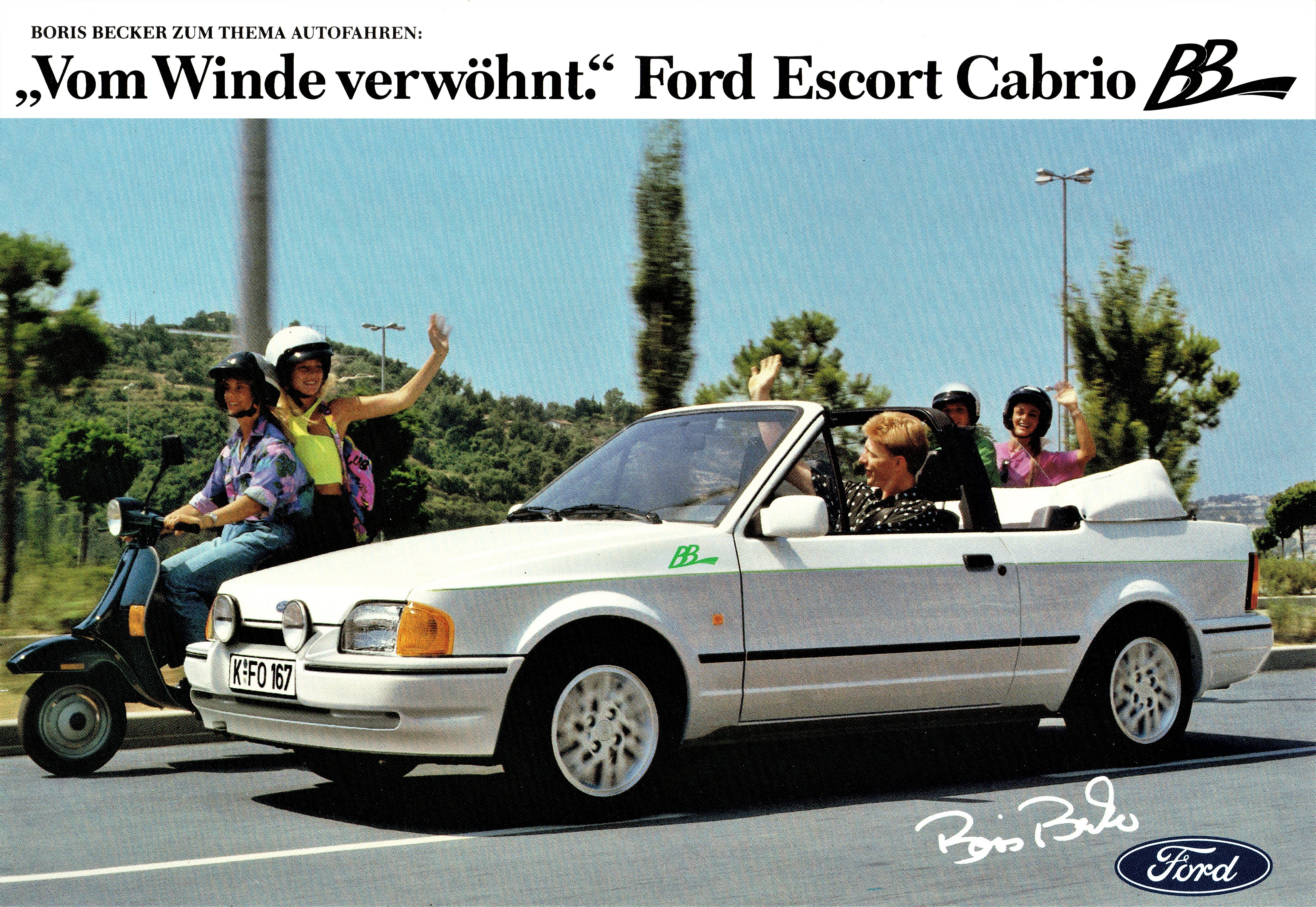In this daytime photograph set in a European locale, a man in a black polka dot shirt is driving a compact white Ford convertible with a European license plate. He is waving to a woman riding on the back of a neon green scooter. The car is prominently displayed with 'Ford' visible in the lower right corner. Behind the man, inside the convertible front of a rollover bar is evident. Another woman, partially obscured by the white car, is also seen waving from the back of another scooter, seemingly directed towards the camera. The scene captures a dynamic moment with the vehicle and scooter heading towards the left of the photo, against a backdrop of trees and shrubbery under a clear sky. The focus is clearly on the car amid a scenic outdoor setting.